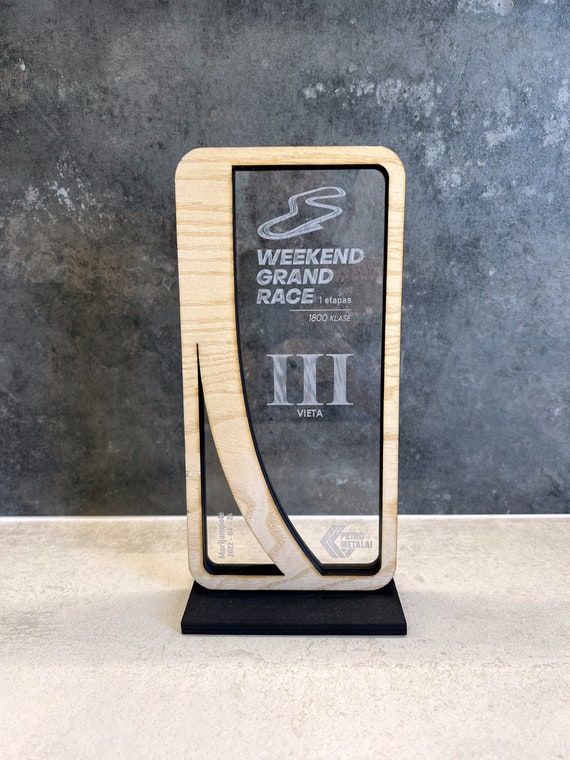The image depicts a detailed digital photograph of a rectangular trophy commemorating a third-place finish in a car race known as the "Weekend Grand Race". The trophy features a sleek wooden pattern frame with two clear, etched glass panels, all standing on a solid black base. The larger glass inlay prominently displays "Weekend Grand Race" in capital white letters, the Roman numeral III, and the word "Vieta," indicating the third-place award. Additionally, there is a detailed engraving of a racetrack above the text, illustrating the race circuit with several twists and turns. In the lower corner, a logo is visible, while the date of the event is etched into the lower left side of the glass. The background consists of a gray marbled wall, and the trophy rests on a smooth white surface. The colors primarily include shades of brown, gray, and hints of silver, contributing to the trophy's sophisticated appearance.